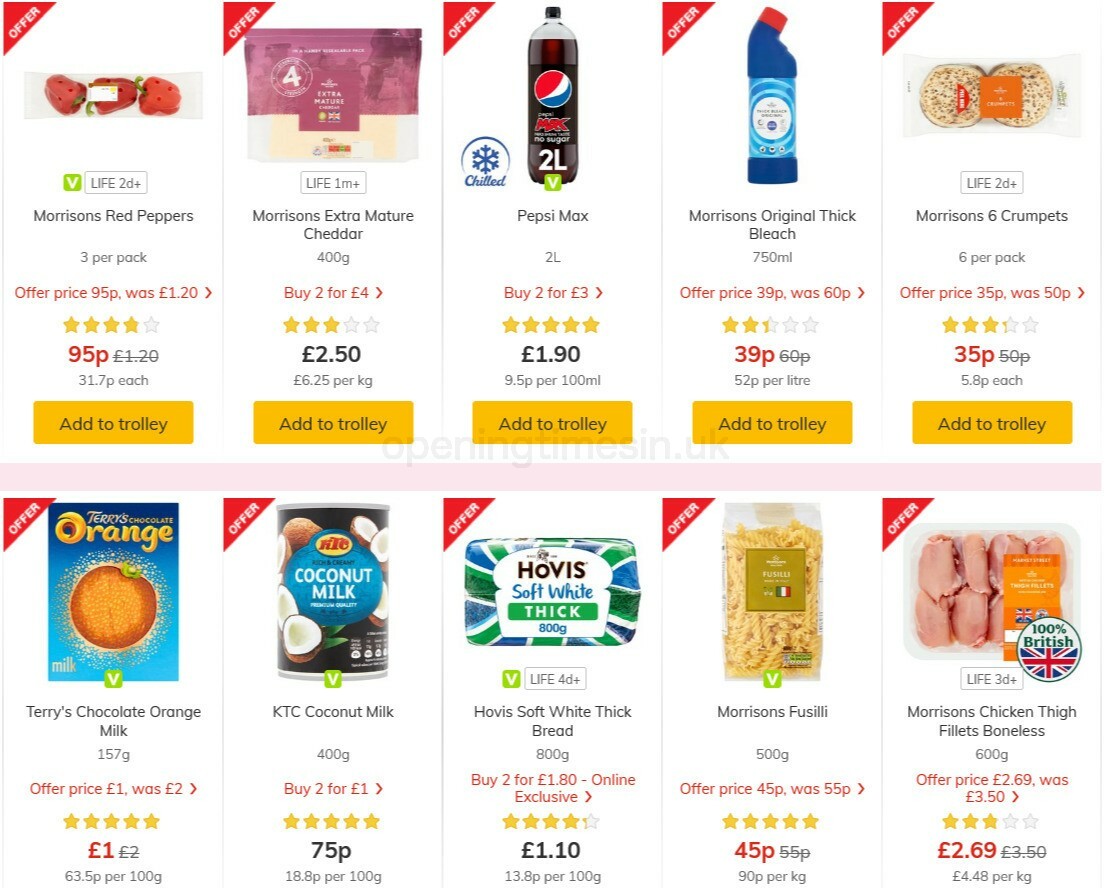The image is a large, horizontal display with a pure white background, likely originating from a computer screen showing various shopping offers. The layout consists of an array of 10 rectangles arranged in two rows of five. Each rectangle features an orange triangle positioned in the upper left corner, marked with the word "offer" in white text. Below this, a detailed depiction of a food item is presented, providing all pertinent information such as the product name, quantity, offer details, rating, and price in pounds or pence. An orange "Add to Trolley" button is present beneath each item, allowing for easy addition to the shopping cart.

### Detailed Descriptions of the First Three Items:

1. **Morrison's Red Peppers**
   - **Quantity**: 3 per pack
   - **Offer Price**: 95 pence (original price 1.20 pounds, now crossed off)
   - **Rating**: 4 out of 5 stars
   - **Additional Info**: 31.7 pence each
   - **Action Button**: Orange button labeled "Add to Trolley"

2. **Morrison's Extra Mature Cheddar**
   - **Weight**: 400 grams
   - **Offer**: Buy two for 4 pounds
   - **Rating**: 3 out of 5 stars
   - **Price per Item**: 2.50 pounds each
   - **Price per Kilogram**: 6.25 pounds
   - **Action Button**: Orange button labeled "Add to Trolley"

3. **Pepsi Max**
   - **Quantity**: 2 liters
   - **Offer**: Buy two for 3 pounds
   - **Rating**: 5 out of 5 stars
   - **Price Per Bottle**: 1.90 pounds
   - **Price per 100 ml**: 9.5 pence
   - **Special Note**: Features a "chilled" icon
   - **Action Button**: Orange button labeled "Add to Trolley"

The remaining seven items follow a similar format with detailed information about the product name, quantity, offer details, ratings, price, and an "Add to Trolley" button. The cohesive structure and clear presentation make it easy for users to compare and select their desired products efficiently.